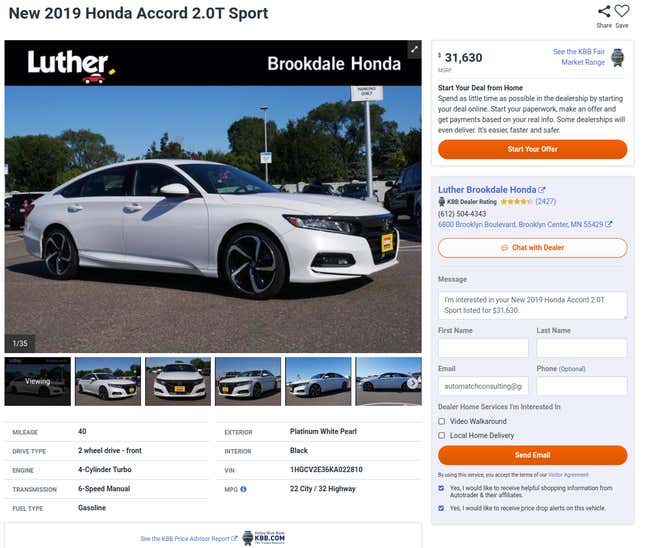**Descriptive Caption:**

This landscape-oriented screenshot captures a detailed view from the official Honda website, showcasing the new 2019 Honda Accord 2.0T Sport. The upper section, with a cream-colored background, prominently displays the model name and features icons for sharing and saving the page on the upper right side.

The content is arranged into two main columns. The left column begins with a black stripe reading "Luther Brookdale Honda" and provides an expandable image section. Below this stripe is a large, clear picture of the Honda Accord parked in a lot with trees and lampposts in the background, tagged "1 of 35" in the bottom left corner. Directly below this main image is a row of six thumbnail images of the car, the first one labeled "viewing." At the far right of this row is a right arrow for additional views.

Further down, detailed specifications are organized into two columns and five rows including: Mileage, Drive Type, Engine, Transmission, Fuel Type, Exterior, Interior, and VIN information.

The right column displays the price "$31,630" prominently at the top followed by "Start your deal from home". Below this is a large, vibrant orange button labeled "Start Your Offer" next to another mention of "Luther Brookdale Honda". There is also a semi-transparent orange button for initiating a chat with a dealer. Further down is a form to fill out personal information and at the very bottom right corner, another large orange button labeled "Send Email". 

The overall layout is well-organized and user-friendly, designed to offer comprehensive information about the 2019 Honda Accord 2.0T Sport at a glance.